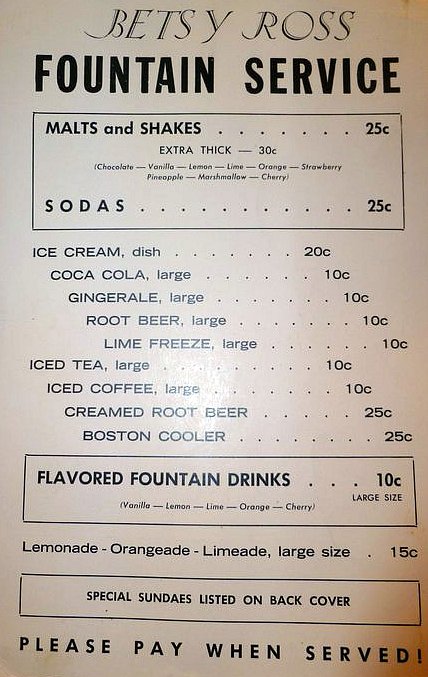This is a photograph or scan of a vintage menu page, featuring black font on a white background. At the top, the menu proudly displays the title "Betsy Ross" followed by "Fountain Service." Below, a neatly drawn black-ink rectangle encloses the text, highlighting various malt and shake options: "Malt and Shakes ... 25 cents" with an additional note for "Extra Thick - 30 cents." 

Further down, the menu lists:

- "Sodas ... 25 cents"
- "Ice Cream Dish - 20 cents"
- Beverages such as "Coca-Cola (Large) - 10 cents," "Ginger Ale (Large) - 10 cents," "Root Beer (Large) - 10 cents," "Lime Freeze (Large) - 10 cents," "Iced Tea (Large) - 10 cents," and "Iced Coffee (Large) - 10 cents"
- Specialty drinks including "Creamed Root Beer - 25 cents" and "Boston Cooler - 25 cents"

Another black-ink rectangle emphasizes "Flavored Fountain Drinks ... 10 cents," with a note mentioning "Large Size" beneath it. 

Below this, additional drink choices are listed: "Lemonade, Orangeade, Limeade (Large Size) - 15 cents." The menu concludes with instructions: "Special Sundaes listed on the back cover" and a polite reminder, "Please pay when served."